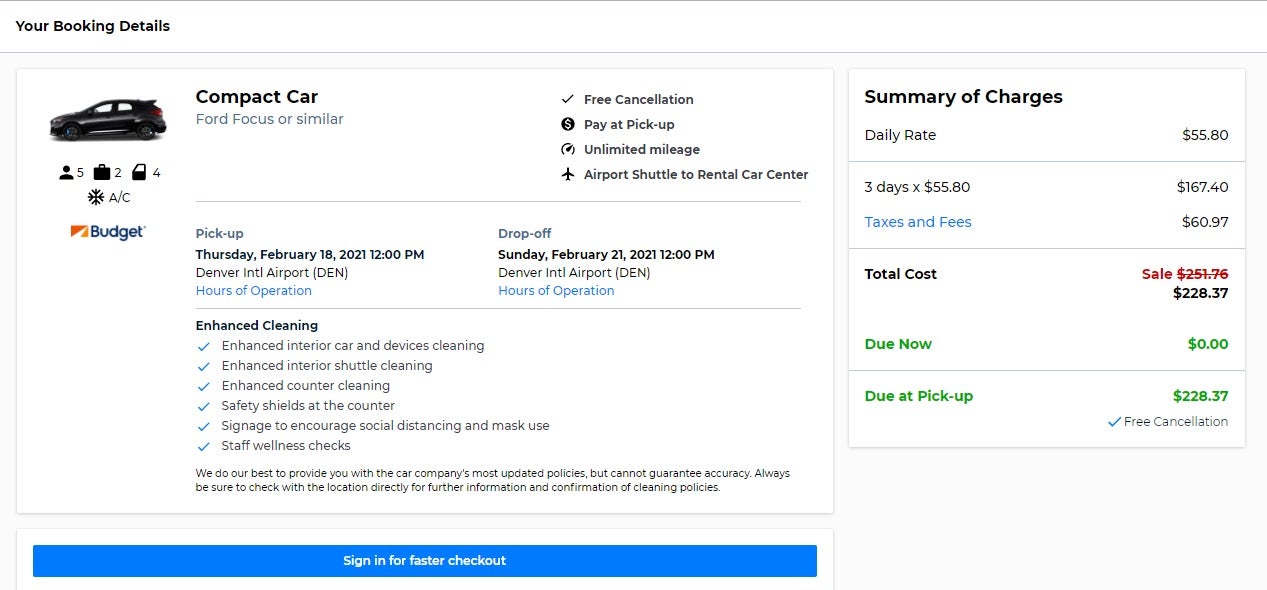**Booking Details: Ford Focus or Similar**

*Vehicle Type*: Compact Car  
*Color*: Black (facing left)

**Rental Features**:
- **Free Cancellation**
- **Pay at Pickup**
- **Unlimited Mileage**
- **Airport Shuttle**: Provided to rental car center

**Rental Period**:
- **Pickup**: Thursday, February 18th, 2021 at 12:00 PM  
  *Location*: Denver International Airport (DEN)
- **Drop-off**: Sunday, February 21st, 2021 at 12:00 PM  
  *Location*: Denver International Airport (DEN)

**Operational Hours**: Matching airport hours of operation

**Enhanced Cleaning Procedures**:
- Deep cleaning of car interiors and devices
- Thorough cleaning of interior shuttle buses
- Enhanced counter cleaning
- Installation of safety shields at the counter
- Signage promoting social distancing and mask use
- Wellness checks for staff

*Note*: We aim to provide the most up-to-date policies from the car rental company, although we cannot guarantee their accuracy.